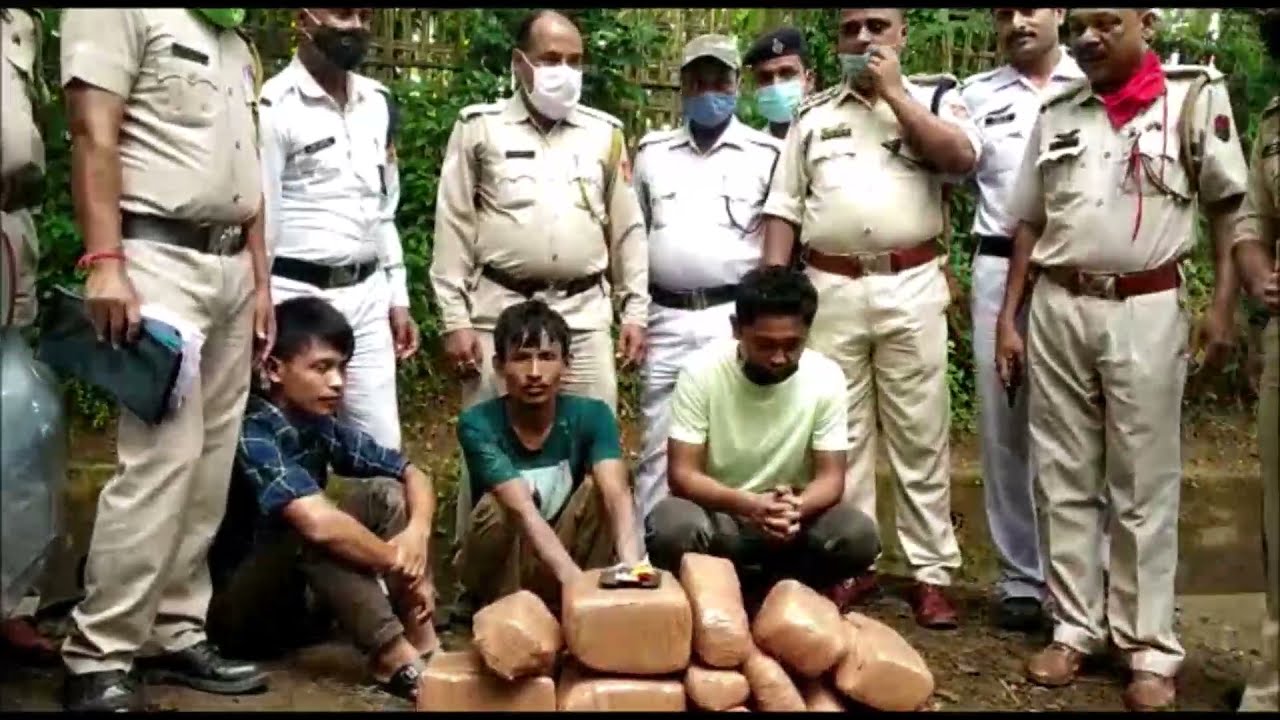The image captures a tense police or military drug bust scenario. At the center are three young men, squatting with forlorn expressions, seemingly arrested for smuggling drugs. In front of them, there is a prominent pile of approximately ten rectangular bricks, wrapped in light brown packaging, suggesting they contain illegal substances like cocaine or heroin. Surrounding the trio are ten men, dressed in tan button-down shirts and matching dress pants, complete with shoulder straps, badges, and name tags. These uniformed individuals are likely police or military officials, most of whom are wearing surgical masks. The scene appears to involve authorities from an Asian or Latin American background, possibly South American, indicating a serious crackdown on drug trafficking activities.